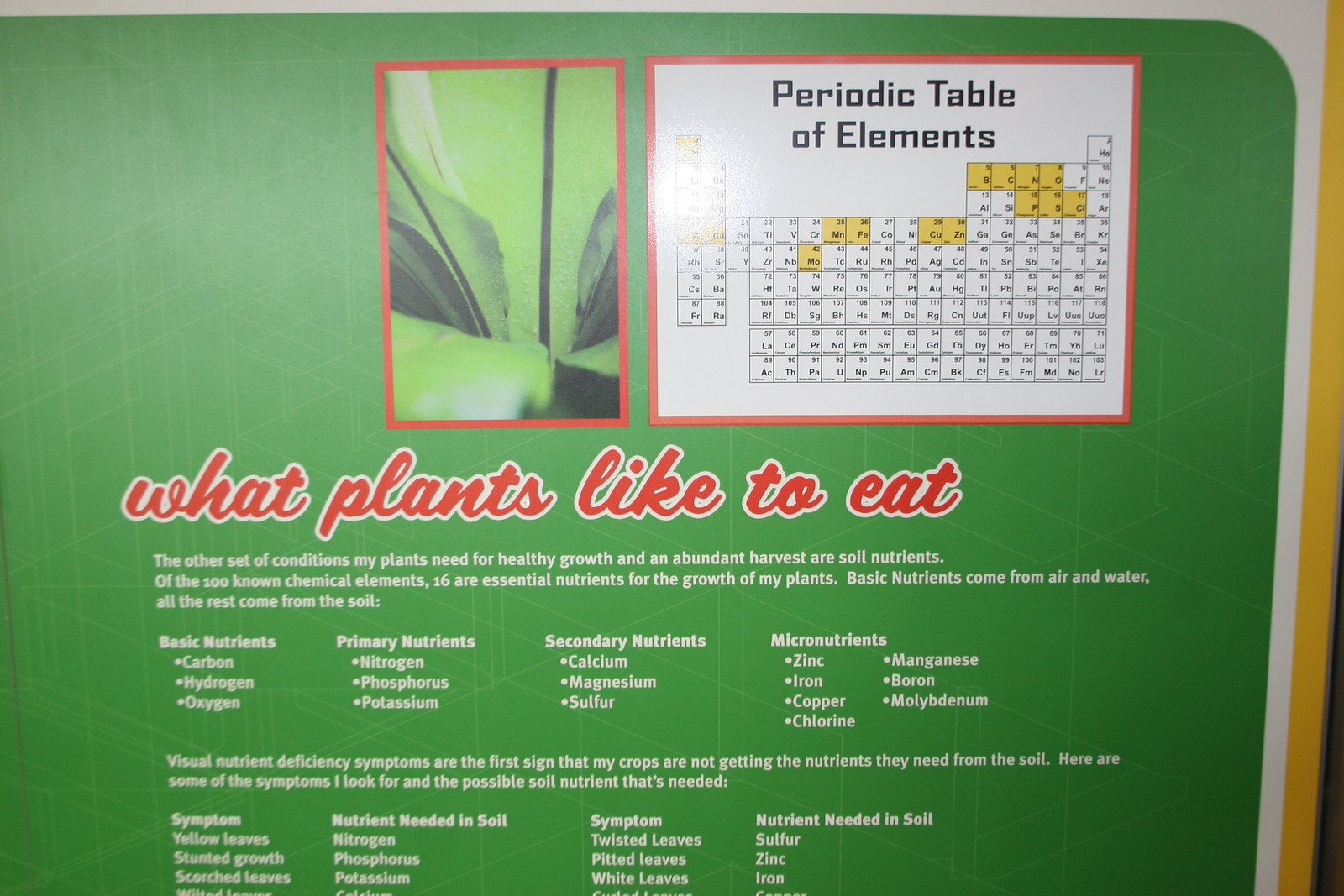The image resembles a digital display or possibly the cover of a textbook, illustrating essential information about plant nutrients. It features a green background with a central red-bordered picture showing a close-up of plant leaves. To the right, on a white background, is the label "Periodic Table of the Elements," with the actual periodic table displayed below in black and white, with some cells highlighted in yellow. Beneath this, in bold red script, is the title "What Plants Like to Eat." Following the title is a paragraph in white font: "The other set of conditions my plants need for healthy growth and abundant harvest are soil nutrients. Of the 100 known chemical elements, 16 are essential nutrients for the growth of my plants. Basic nutrients come from air and water. All the rest come from the soil." Below, various categories of nutrients are listed: basic nutrients, primary nutrients, secondary nutrients, and micronutrients, each followed by a bulleted list of elements such as carbon, hydrogen, oxygen, nitrogen, phosphorus, and potassium. At the bottom, another paragraph reads, "Visual Nutrient Deficiency Symptoms: The first sign that my crops are not getting the nutrients they need," followed by a table. The table contains column headings such as "Symptom" (e.g., yellow leaves) and "Nutrient Needed in Soil" (e.g., nitrogen), providing a guide to identify and address nutrient deficiencies in plants.